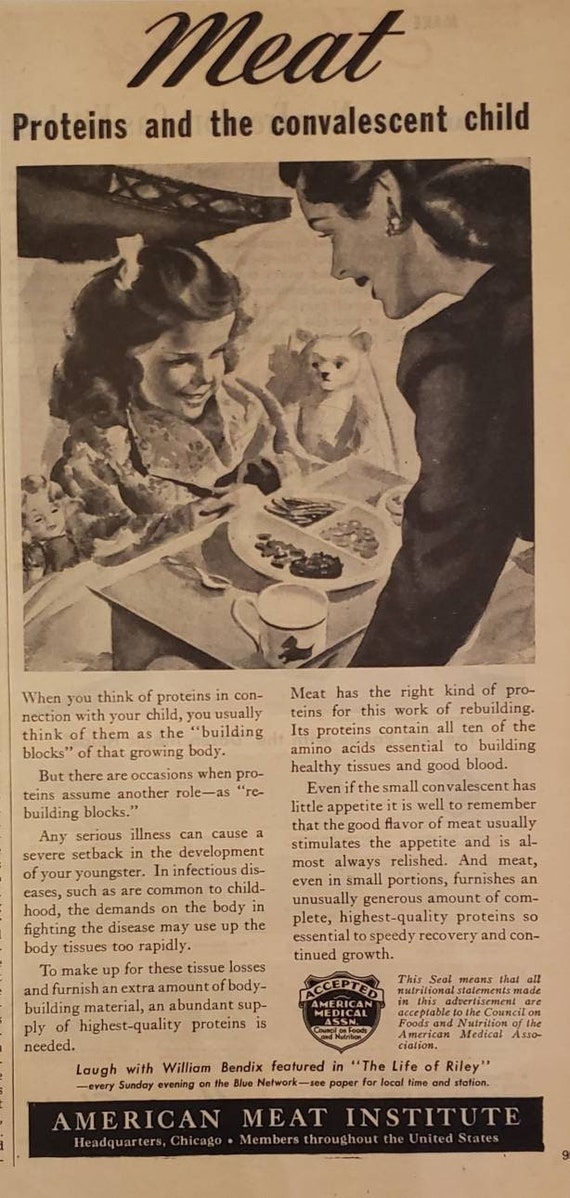The image is an aged black-and-white advertisement, likely a clipping from an old newspaper or magazine, with a backdrop that has turned a brownish color over time. At the top, in cursive with a prominent capital "M," is the word "Meat." Below it, in printed text with a capital "P," are the words "proteins and the convalescent child."

The central part of the image features an illustration of a mother serving breakfast in bed to her daughter. The mother, dressed in a black top with long, dark hair reaching her shoulders, is smiling down at the young girl. The daughter, who appears to be recovering from an illness, is seated on a bed with a white pillow and covered with a white blanket. She has long, dark hair adorned with a bow tie. To her left and right are her stuffed animals and dolls. On the tray the mother is holding, there are three sections containing various vegetables and foods, a plate with some items resembling peas, and a white teacup with a spoon.

Below the image, on either side of the illustration, are several paragraphs of text. Embedded within the text is a small shield logo with the word "Accepted" written on it, possibly followed by "American Medical." At the bottom of the image, in a black strip with white text, are the words "American Meat Institute, headquarters Chicago, members throughout the United States."

The overall impression is that of a nostalgic advertisement promoting the benefits of meat and proteins for the recovery of sick children, with a detailed and tender depiction of a mother caring for her daughter.